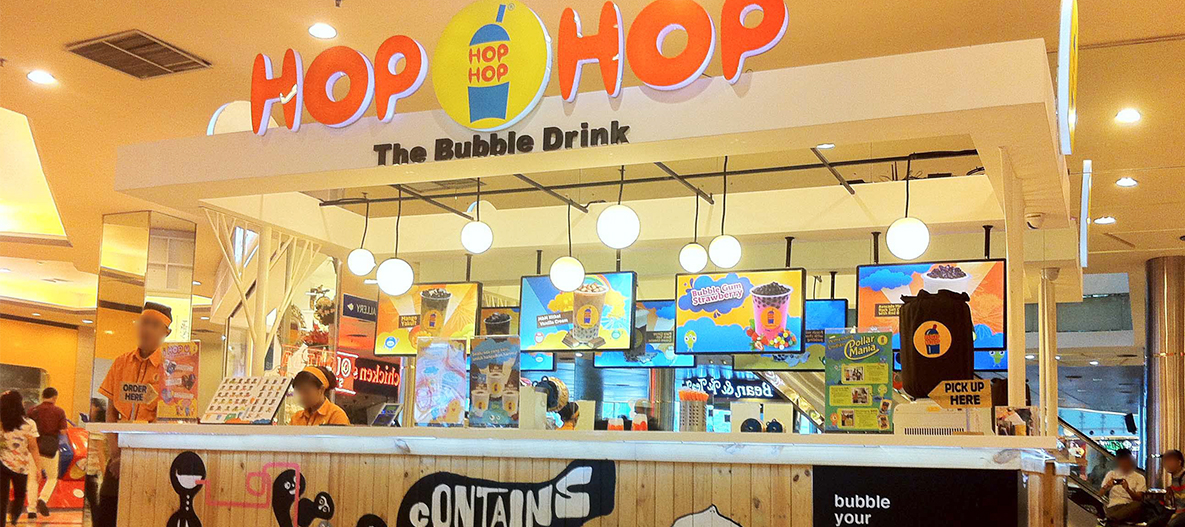The photograph captures a vibrant drink stand situated in the middle of a concourse, likely in a bustling mall. The counter is constructed from light brown wood panels with a sleek white countertop. Above it, a prominent signboard reads “Hop, hop, the bubble drink” in orange letters, flanked by a blue circle logo depicting a plastic cup with the words “Hop, hop.” Two employees, dressed in matching orange polo shirts and headbands, can be seen serving customers—one is standing while the other is seated behind the counter. Multiple colorful LED screens behind them showcase an array of beverages. The stand, with its white rooftop and visible air conditioning vent in the top left corner, is surrounded by the dynamic environment of the mall, complete with recessed lighting and bustling shoppers.